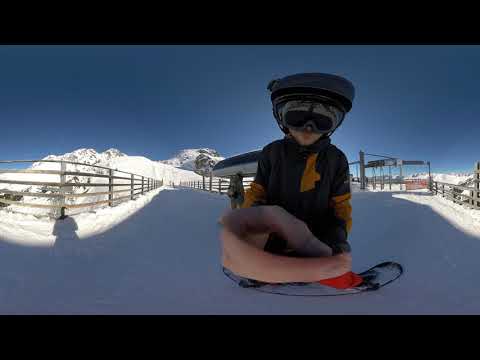In this point-of-view photograph of a snowboarding scene, the person taking the picture is visibly stopped on a snow-covered slope. The sky above is a light gray, devoid of clouds, contrasting with the distant mountains blanketed in white snow and speckled with rocky gray outcroppings. In the immediate foreground, the snowboarder's black-gloved hand holds the camera, focusing on their feet strapped into a black snowboard. Their attire includes bright orange pants and a distinctive black jacket with yellow sleeves and a yellow front. The snowboarder is also equipped with a black helmet and gray-rimmed black-lensed goggles. Flanking both sides of the person are wooden railing fences, adding to the wintry aesthetic. While the picture predominantly showcases the snowy landscape, a wooden structure is faintly visible in the background, and the snow-covered ground extends beneath them, enveloped in the cool hue of this serene vista.